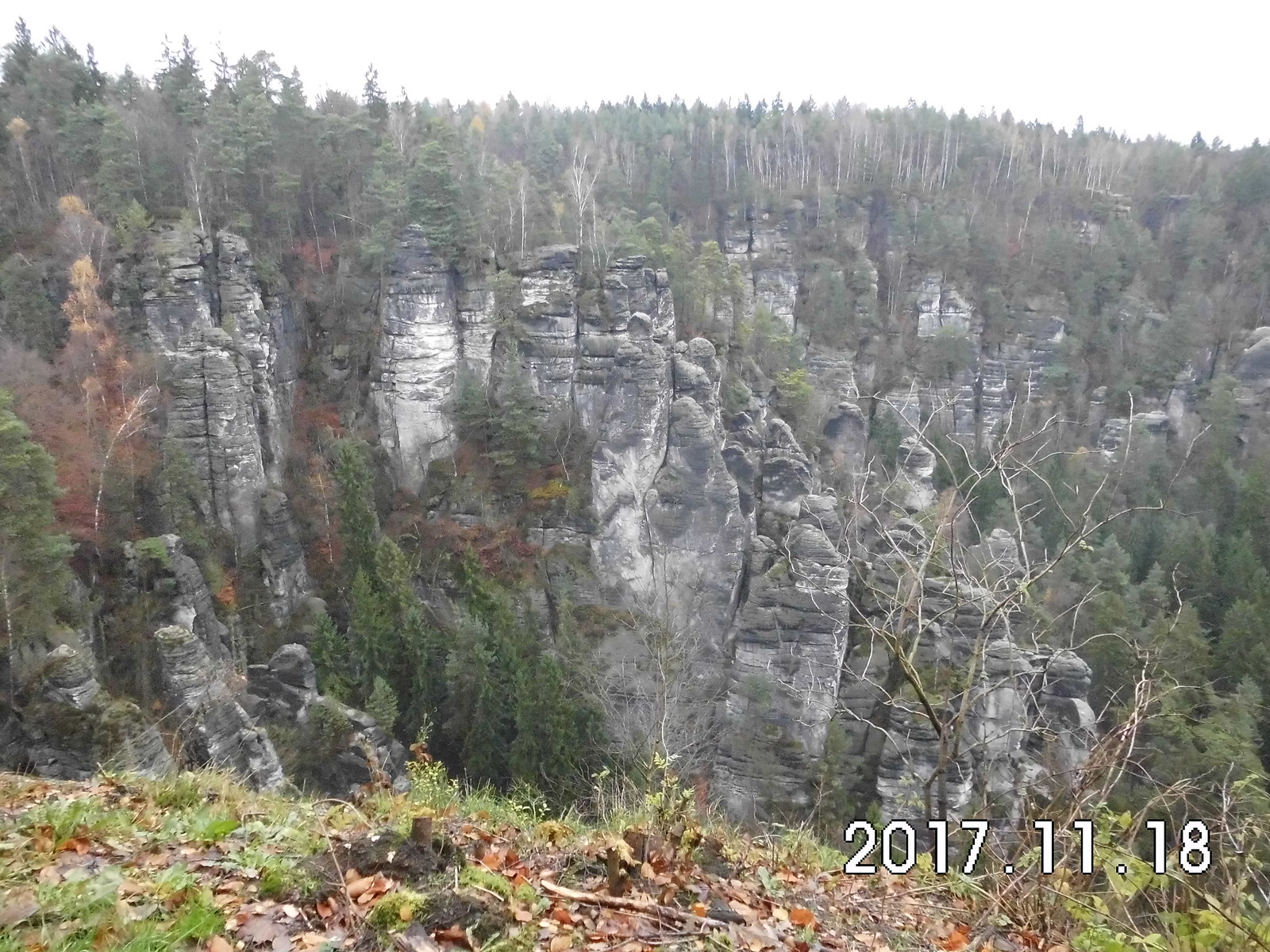This photograph, taken on November 18, 2017, captures a striking view of a valley dominated by tall, thin cliffs or stone pillars, which are grayish and marked by age. The landscape features a mixture of dark green pine trees and colorful foliage, including orange and red trees, growing between and on these unique formations. The foreground reveals dried leaves, deep brown dirt, and varying shades of green, brown, and orange shrubbery. The sky above is a flat, ambiguous shade, appearing either white or gray, devoid of color. There is no text or people present in the image, emphasizing the natural beauty and solitary grandeur of the scene.